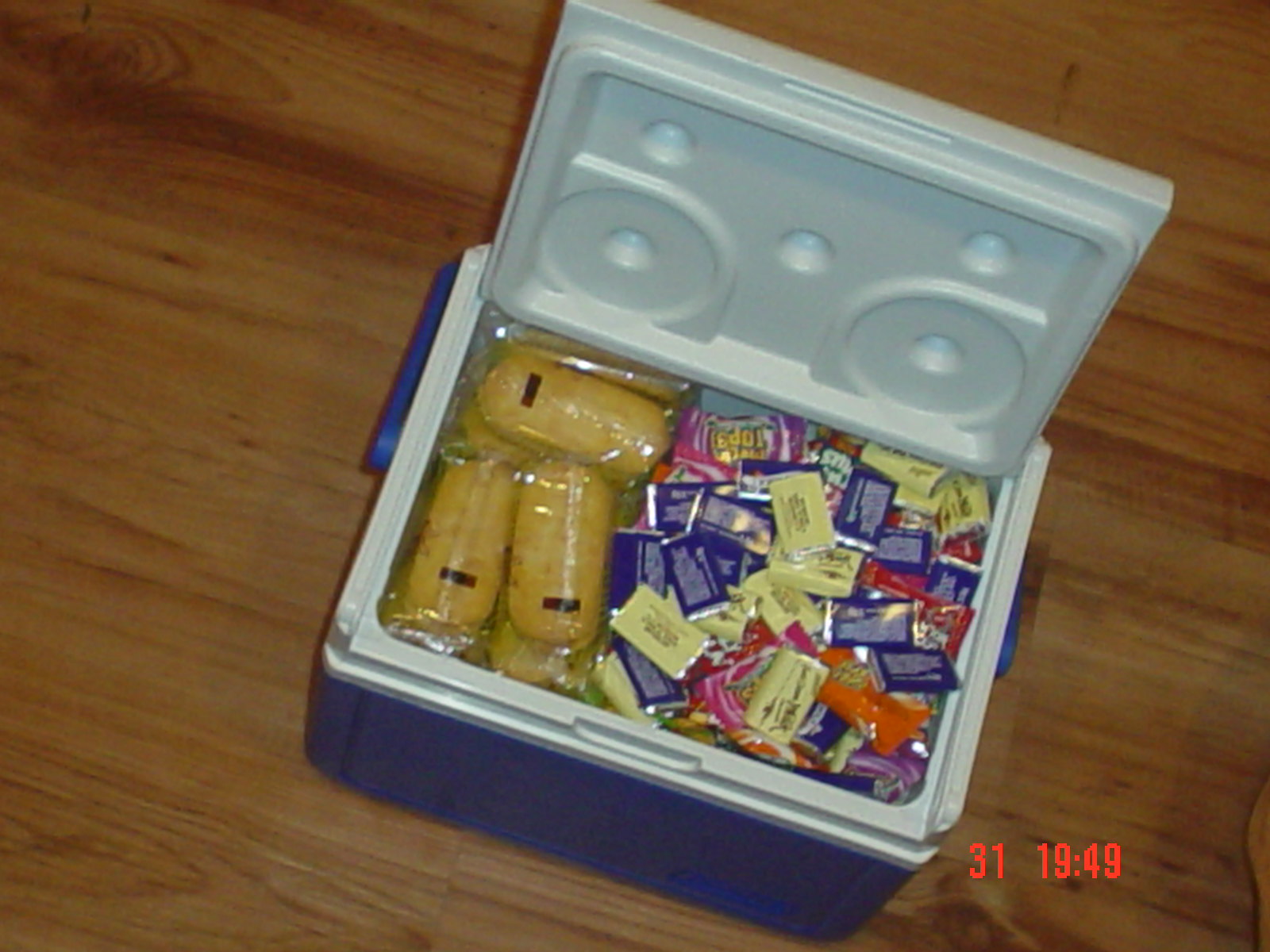A blue and white cooler with a blue handle is sitting on a light brown wooden floor. The cooler, which has an open lid, is filled with snacks and treats. On the left side, a pile of individually wrapped Twinkies, recognizable by their light brown round appearance in clear wrappers, takes up one-third of the space. The right two-thirds are occupied by an assortment of miniature candies and chocolates, each wrapped in an array of colorful wrappers, including blue and silver, yellow and silver, orange, and pink. The bottom right corner of the photo features a red time stamp that reads "31 19:49." The cooler, reminiscent of those used in the mid-2000s, appears slightly aged, adding a nostalgic touch to the image.